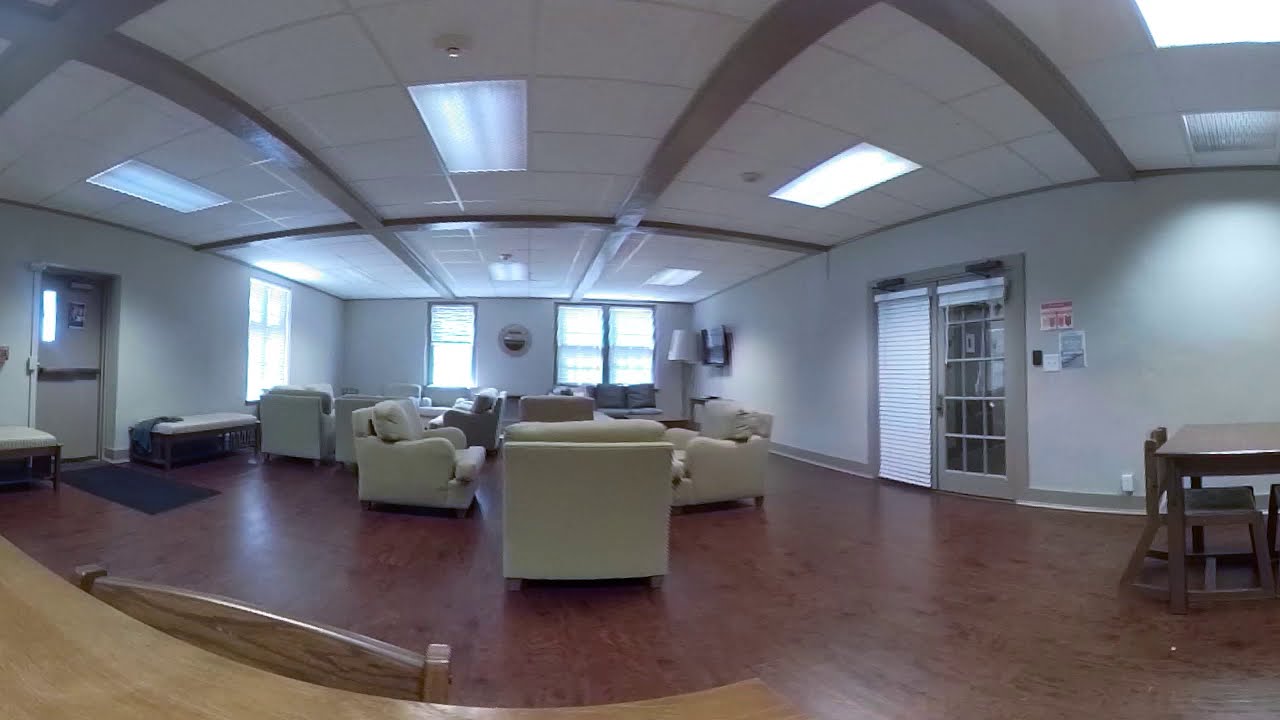The image depicts a spacious room with white walls and an acoustical tile ceiling featuring dark stained oak beams and fluorescent lighting panels. The room has beige and white furniture predominantly arranged towards the center, including multiple sofas, chairs, and at least one table with a chair pushed into it. The flooring appears to be either man-made wood or solid wood. Large windows are visible on two sides, allowing natural light to flood the space, and there are doorways on the left and right walls. The room seems to be an indoor space, possibly a commercial setting such as a waiting room or a church basement, given its furnishings and overall layout. The scene is likely set during the daytime, indicated by the natural lighting. Various colors are present in the image, including light brown, dark brown, black, white, gray, tan, red, and light blue, adding a subtle vibrancy to the otherwise neutral-toned room.